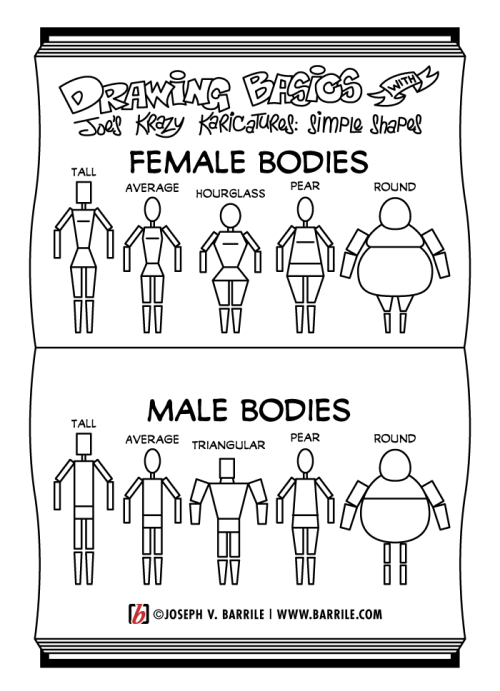This detailed black and white image appears as an illustrated poster or open book page titled "Drawing Basics with Joe's Crazy Caricature Simple Shapes." The design prominently features simplified, line-drawn representations of various body types for both females and males. For female bodies, the types displayed are tall, average, hourglass, pear, and round. Correspondingly, the male bodies shown include tall, average, triangular (with notably blocky shoulders), pear, and round. The figures resemble wooden posing mannequins often used in drawing. The entire composition takes up most of the vertical layout of the image, with a clear and minimalistic aesthetic, focusing purely on the essential shapes without detailed features or colors beyond black and white. At the bottom, the image includes the text “Copyright Joseph V. Barilli” along with the website “www.barilli.com.”